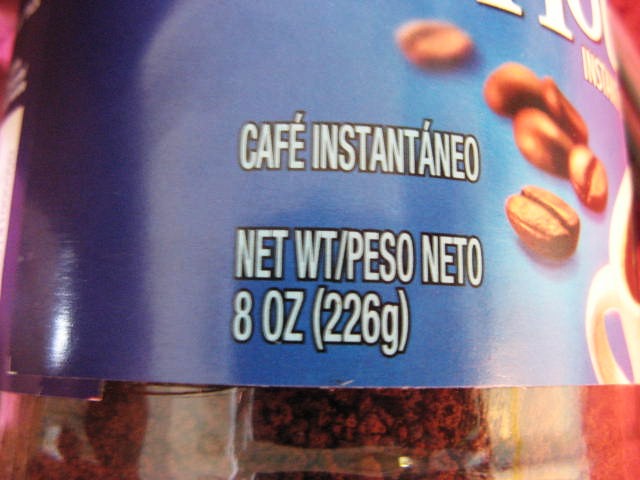Close-up view of an instant coffee product label. The image prominently features the side of a clear plastic container, filled with dark coffee granules visible through the transparent material. The brand name, written in large, bold letters, indicates that this is a café-style instant coffee, with the labeling done in Spanish. The label includes details about the product's weight, provided both in pesos and English measurements, showing ounces and grams. Scattered coffee beans illustrate the aromatic appeal of the coffee, adding a decorative touch around the lettering. A large logo or brand name is partially visible in the top right corner, just outside the main focus of the label. This detailed label visually communicates key product information, ensuring clarity for the consumer.